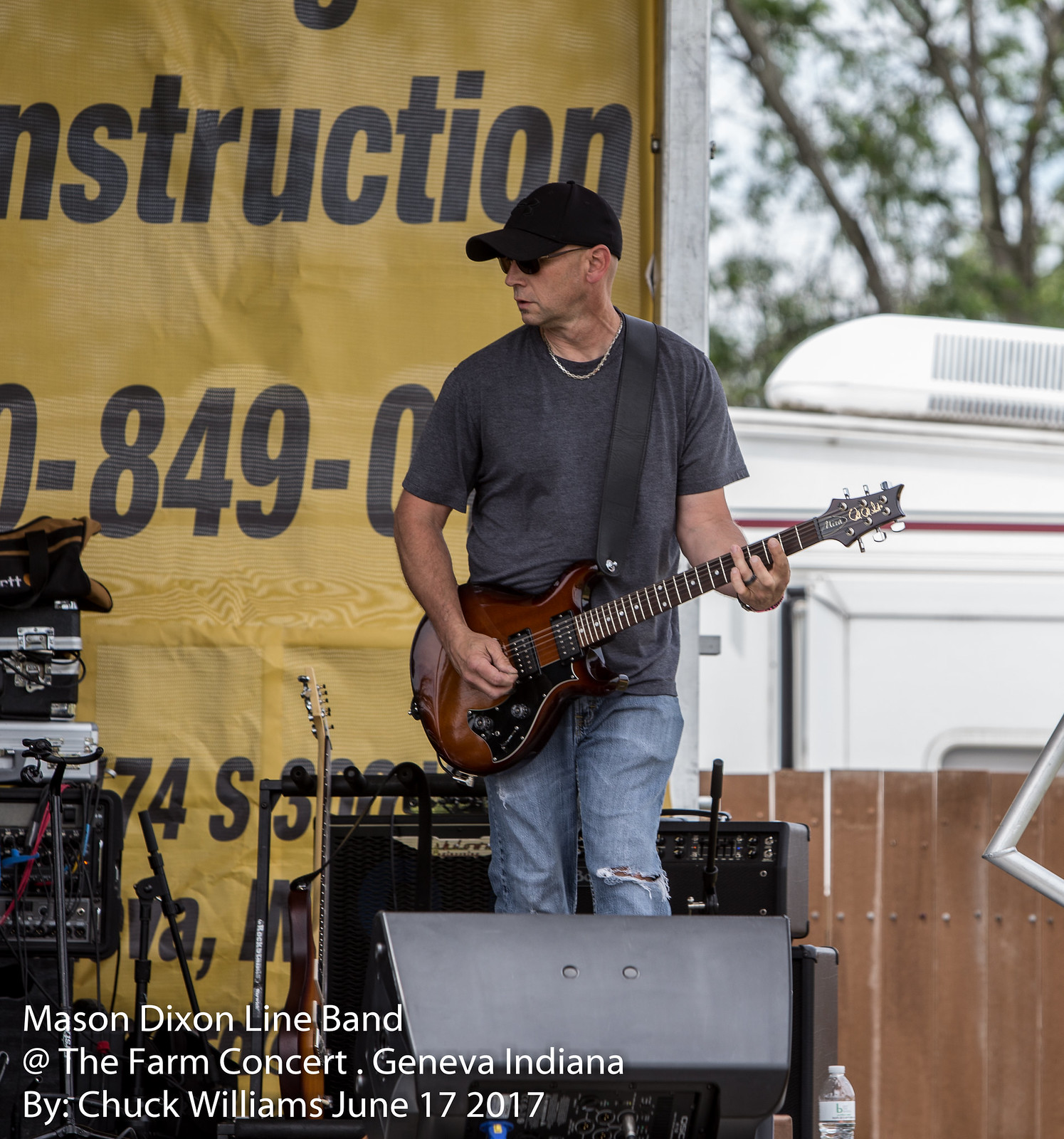This image captures a man performing at a concert, exuding a charismatic presence on stage. He is adorned in a black baseball cap, sunglasses, a gray t-shirt, a silver chain, and blue jeans with rips at the knees. The musician is passionately playing a brown electric guitar, its body bearing the rich hue of dark, burnt orange wood. Glancing to his right (our left), he stands before an array of electronic music equipment, including a speaker and another guitar on a stand directly behind him.

In the background, a partially visible banner, with only the first and second 'N' of "construction" and parts of a phone number (8, 4, and 9) discernible, hints at a sponsorship or advertisement. The backdrop also contains an illegible address at its bottom. Behind the stage on the right, there is a fence with a camper parked behind it, contributing to the rustic concert ambiance. A distinct yellow backdrop frames the scene.

The lower left corner of the image features text crediting the photo: "Mason Dixon Line Band at the Farm Concert, Geneva, Indiana by Chuck Williams, June 17, 2017." The clear weather and the enthusiastic crowd reflect the lively atmosphere of the farm concert.